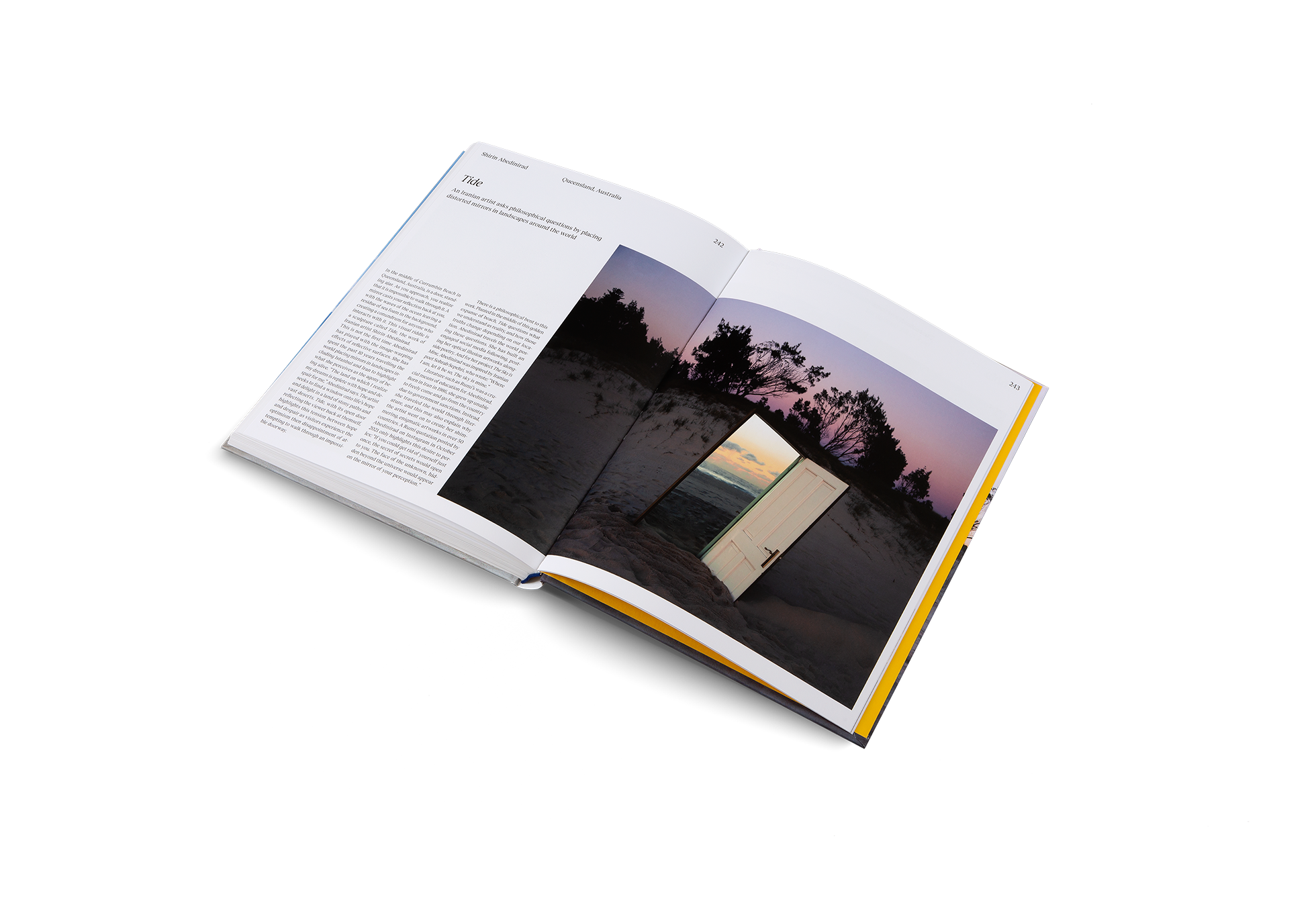The image depicts a modern, square-format color photograph of an open book, angled with the left side facing the top left and the right side facing the bottom right, spread wide on a surface. The pages, predominantly white, reveal a sophisticated, clean-cut serif typeface that suggests a contemporary design. There is a vivid full-color photograph spread across the right page and extending into the left page, showcasing a surreal outdoor scene. The scene features light brown desert sand with silhouetted trees and bushes against a sunset sky in hues of lavender and pink. In the foreground, a striking, white open doorway is Photoshopped into the sand, creating a sci-fi-like portal to a coastal scene with the ocean and a blue-pink sky. This doorway, embedded in the sand, seems to offer a passage to another dimension, blending realism and fantasy. On the left page, there are two paragraphs of black text and a bold header, 'TIDE,' in the top left corner. The text is illegible due to distance. The background is white, making the book appear to float, enhancing its modern aesthetic.